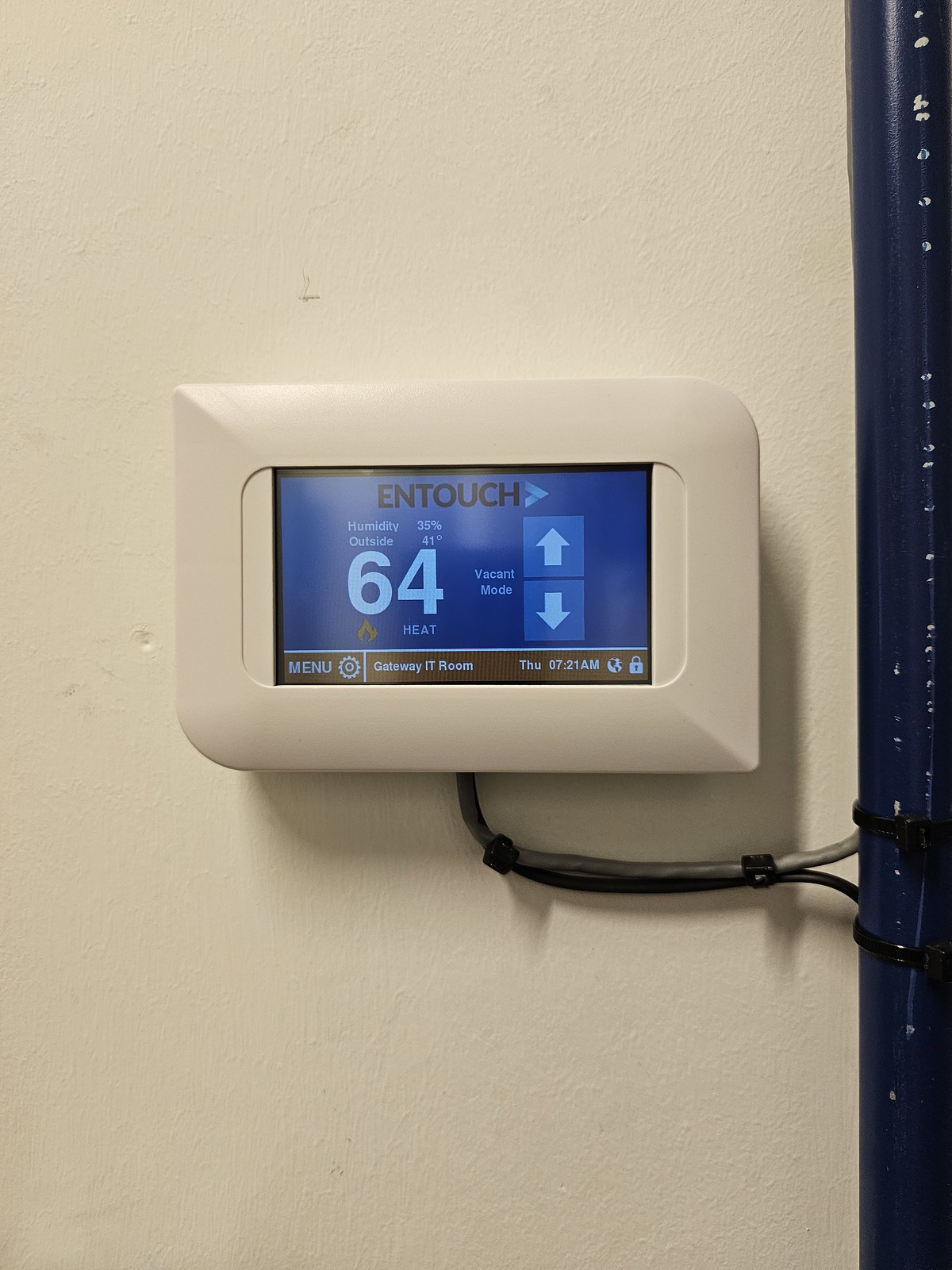In the image, the central feature is a sleek digital display showcasing the text "In Touch" in bold black letters. The display indicates various environmental readings, such as "Humidity: 35%" and "Outside: 41 degrees." It also shows "64 Heat" and mentions it is in "Vacant mode." Navigation arrows, one white pointing up and another pointing down, flank the readings. Additionally, there are blue boxes on the interface.

Behind the display is a white rectangular box connected to a pole on the right by a cable. The background wall is a soft beige color. The screen also highlights options such as "Menu" and "Dehumidity," and features a gear icon, indicating settings or configuration options. 

The caption mentions the "Gateway IT Room" and notes the time as "Thursday 7:21 a.m." Also present are a globe icon and a lock symbol, possibly indicating security or connectivity status. Below the main display, there is an orange panel set against a blue background. On the right side, wires lead to a tube, suggesting a connection to an AC unit. The overall scene is dominated by a cool, tech-savvy interface set against a white backdrop.